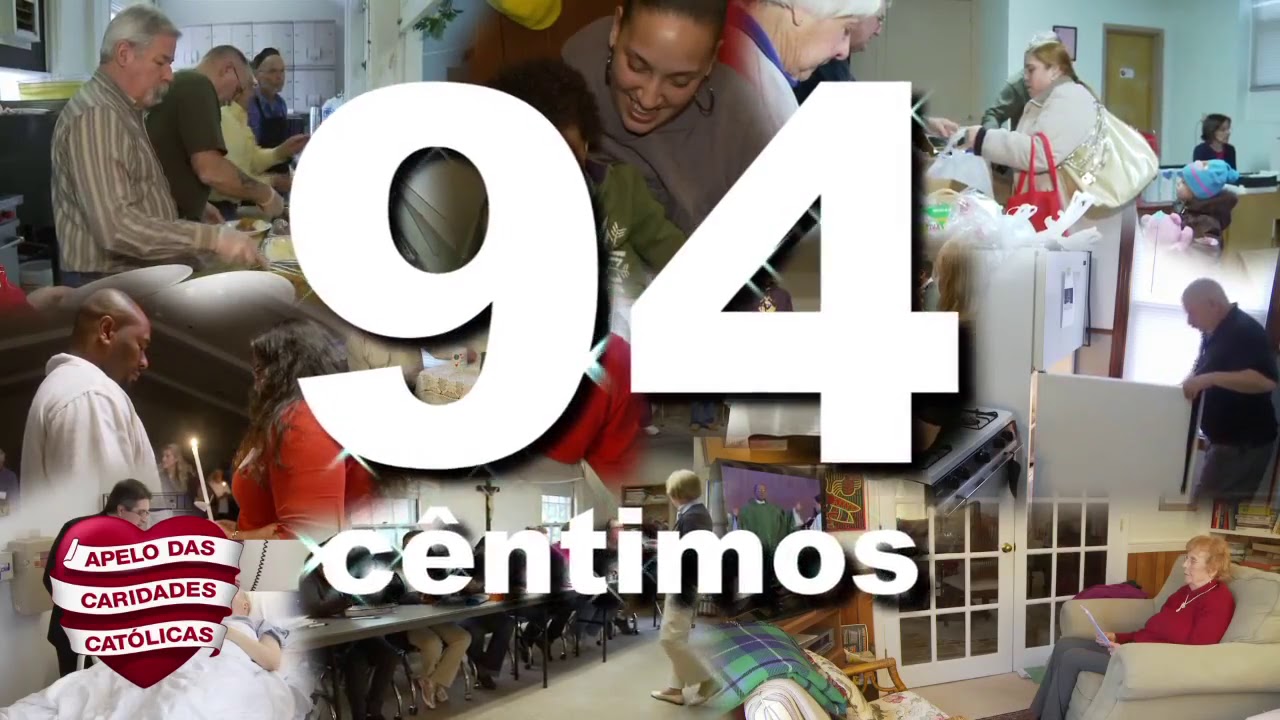This composite image, originating from a Spanish-speaking country, is densely packed with various photographs, overlaid with the prominent white text “94 céntimos” with a shadow effect, positioned centrally. At the lower left corner, a heart shape bears the inscription “Apelo das Caridades Católicas,” suggesting an appeal from Catholic Charities.

In the upper tier of the collage, starting from the left, we observe three older gentlemen possibly eating at a buffet, engrossed in their meals. Moving to the center, a middle-aged individual, whose gender is indistinct, overlooks a smiling companion. Adjacent to this is an older woman, her gaze directed downward, amid bags of items, with a young woman sporting a ponytail and a heavy jacket in the background. The upper right segment reveals a woman at a desk, situated next to a door and beneath a window.

The lower tier commences on the left, behind the heart-shaped overlay, where a person lies in a hospital bed attended by another individual. In the middle, there's a dark-skinned man, potentially a priest, holding a lit candle and engaging with a woman in a red top. This scene is partially obstructed by the numbers 9 and 4. Below the heart, a long table hosts numerous people, though their identities are obscured by the text. Finally, in the lower right corner, an elderly woman with short red hair sits comfortably in a lounge chair, gray slacks on, possibly reading a book or a tablet, in a room with French doors and beige carpeting.

Overall, the composite image evokes a sense of community and care, fitting for a charitable appeal, blending scenes of daily life, support, and interaction within a Spanish-speaking context.